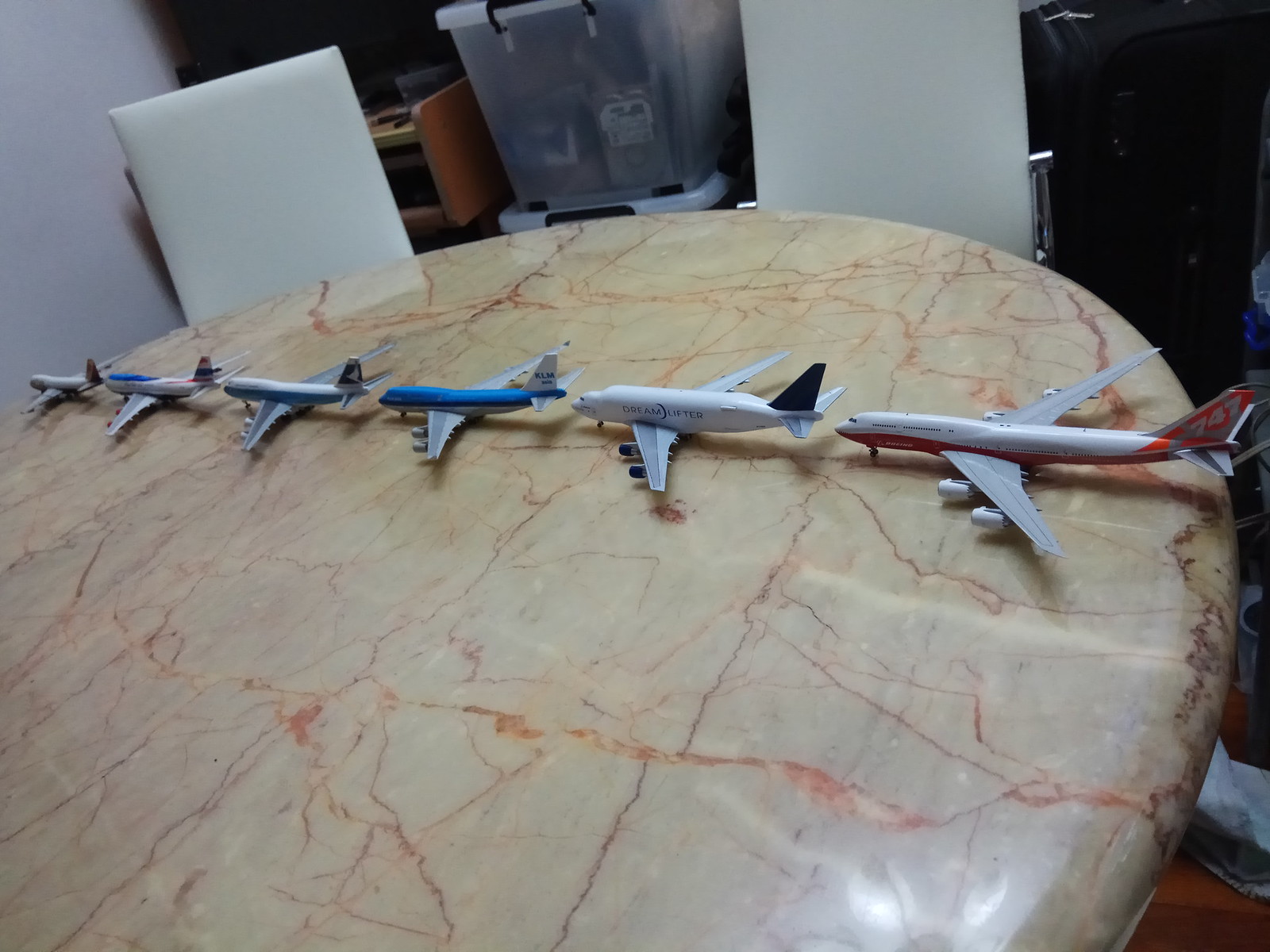The image features a large, round tabletop which appears to be made of synthetic material resembling marble, with a beige and brown color scheme, highlighted by dark brown and rust-colored superficial crack patterns. Positioned neatly across the table are six model airplanes, arrayed in a line facing left. These airplanes are designed to mimic commercial airliners with realistic markings and color schemes. The largest plane is on the far right, marked “747” on its tail and has a red bottom and silver wings. Next to it is a white plane with a blue fin and gray wings labeled "Dreamlifter." The third one is blue on top and white on the bottom, with “KLM” written on its tail. Following it, there is another plane that is white on top with some blue on the bottom. The fifth plane features blue coloring with a red and blue fin. The smallest plane, on the far left, is predominantly white. Behind the table, there are white chairs and a background cluttered with plastic storage bins filled with various items, as well as possible hints of furniture such as a cabinet and possibly some silver candlesticks or lamps. The layout and positioning of the planes, as well as the details of the table, take up the majority of the image.